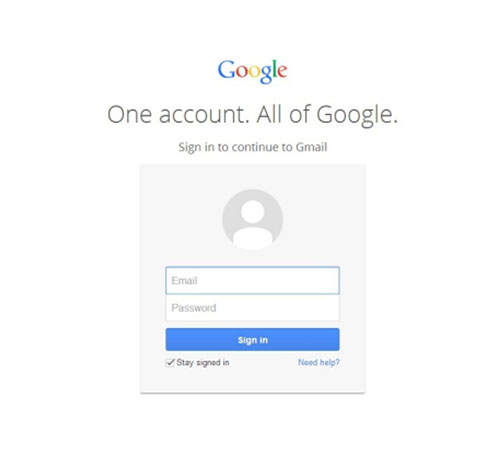The image depicts a Google-powered website for logging into Gmail. At the top, the colorful Google logo is prominently displayed. The 'G' is blue, the first 'O' is red, the second 'O' is gold, the 'G' is blue again, the 'L' is green, and the 'E' is red. Directly below the logo, in black (appearing more like gray) text, it reads: "One account. All of Google."

Beneath this, smaller text instructs users to "Sign in to continue to Gmail." There is a gray box featuring a generic round insignia of a person with a white outline. This imagery represents the user's profile photo placeholder. This box contains an email field that is highlighted in blue, indicating where users should enter their email address. Below the email field, there is a white box designated for the password.

A blue button labeled "Sign in" in white text is located under the password box. To the left of this button, there is an option to "Stay signed in" next to a checkbox, with the text appearing in black or gray. On the right side, the phrase "Need help?" is displayed in blue next to a question mark.

The remaining background of the website is entirely white, except for the login elements, which are housed within their respective boxes.